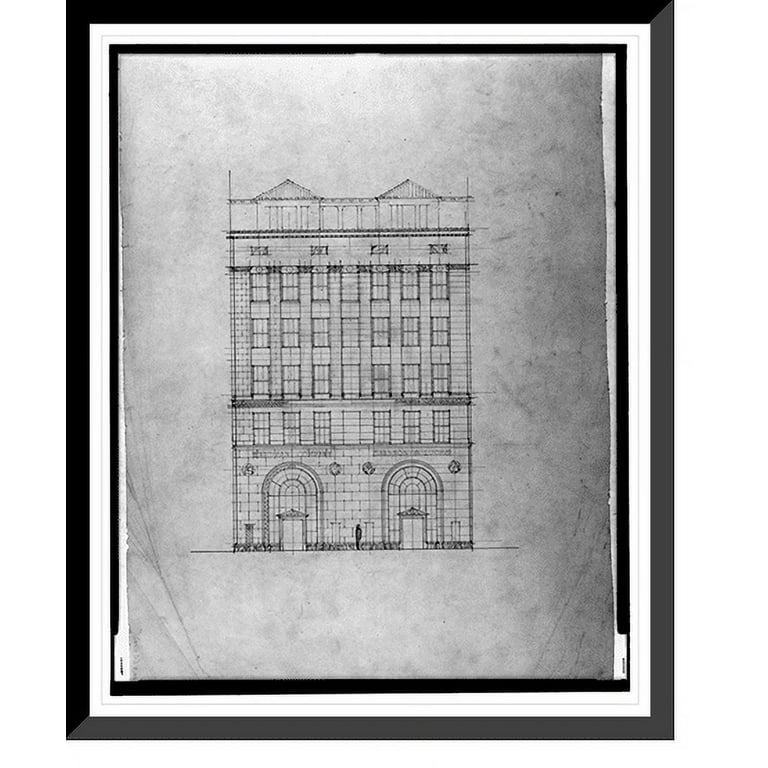The image showcases a detailed architectural drawing of a potentially historic six-story building. The illustration is framed with a black outer frame, followed by a white strip, and another inner black border, which encases the paper. The building features two arch doorways at the bottom, flanked by two doors on either side. Above the doorways, there is a row of windows, followed by three more rows of windows ascending the structure. At the very top, there are two small penthouse-like units with roofs that peak to a point. The scene is devoid of any background or surrounding elements, focusing solely on the building which may hint at a preserved or antique quality. The drawing is in black and white and does not include any labels or signatures to identify the building or its purpose. A small figure of a person is visible standing next to the entrance, emphasizing the scale of the structure. The lines in the drawing suggest the building might be constructed from masonry blocks, but the exact materials remain unclear.